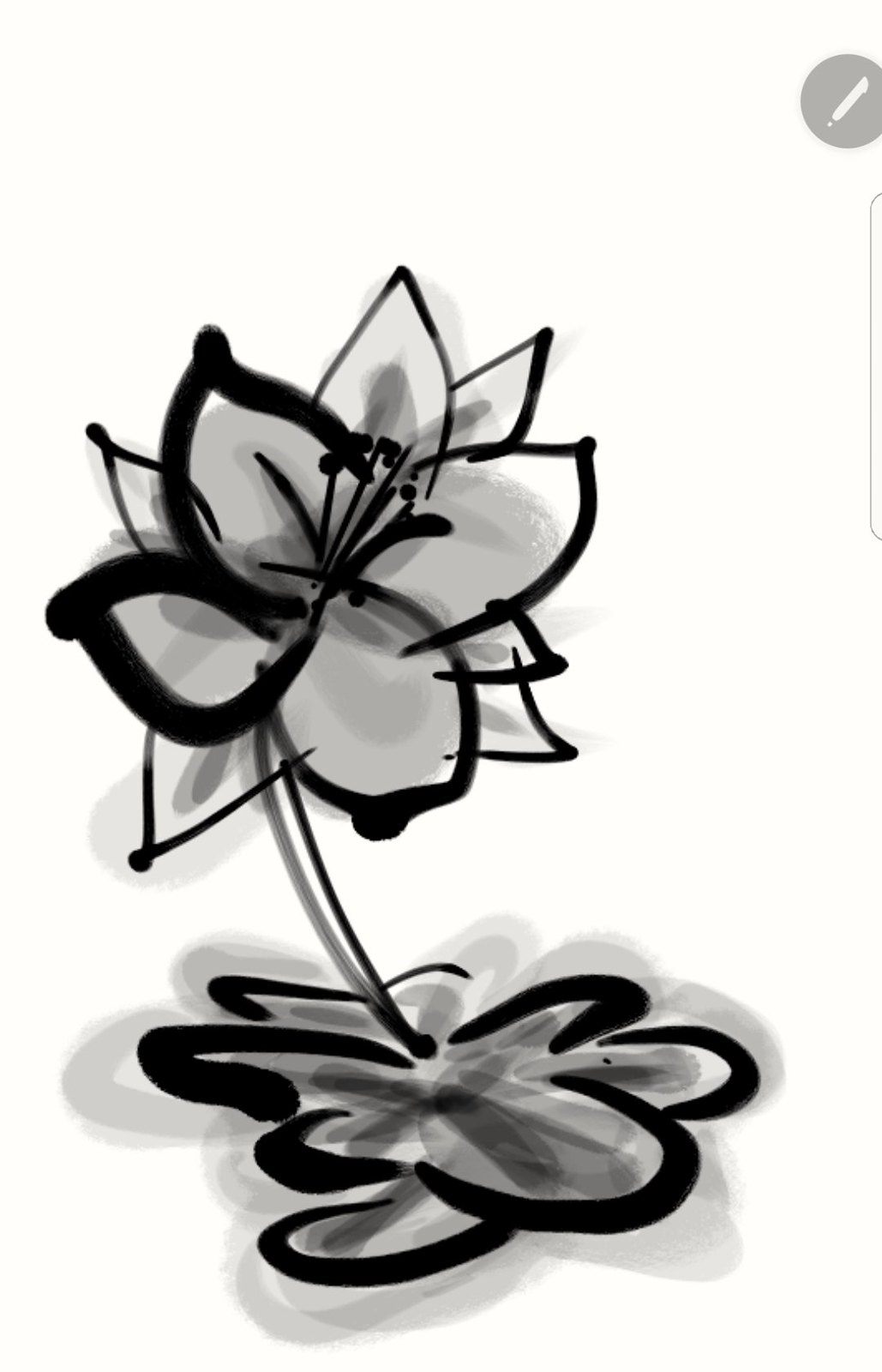The image features a digitally-rendered sketch of a flower with an all-white background, possibly created on a phone as indicated by the subtle icon of a white pen on a gray background in the upper right corner and a strip of a white box on the right side. The flower itself bears a strong resemblance to a hibiscus, with many petals and a somewhat left-leaning stem but a bloom that arcs toward the right. It is outlined in thick black lines and filled with varying shades of gray. The petals are scallop-shaped and arranged in a circular fashion. The flower's stymons extend from the center, topped with small black balls of pollen. Below the flower, there is a shadow, also rendered in shades of black, gray, and white, adding depth to the monochromatic artwork. There is no text and no other colors present in the image, which emphasizes the detailed and textured rendering of the flower and its shadow.